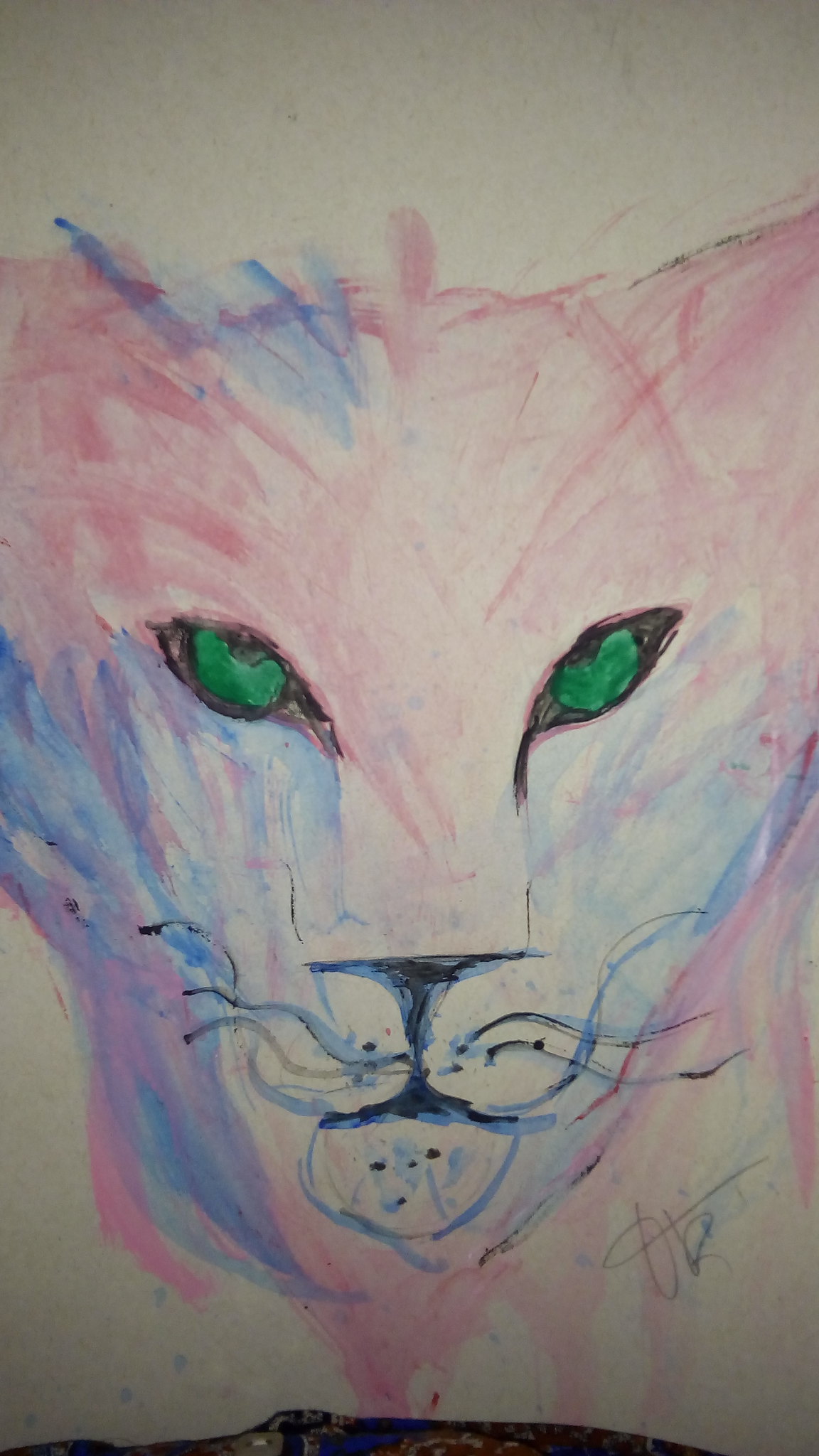This hand-drawn artwork depicts a tiger with vivid green eyes and clearly defined black pupils, gazing upwards with an expression of curiosity. The tiger's head, primarily in shades of pink, is drawn on manila paper, but the tips of its ears are cut off, leaving them unseen. An intricate interplay of pink and blue shading defines the head and face, with blue accentuating the top portion as well as the jawline down to the chin. The tiger’s nose is depicted in black, with a blue undertone, and is surrounded by detailed dots indicating the whisker roots, which can also be seen on the chin. The artist has signed the piece in the lower right-hand corner, and there is an indistinct black mark at the bottom, the nature of which is unclear.